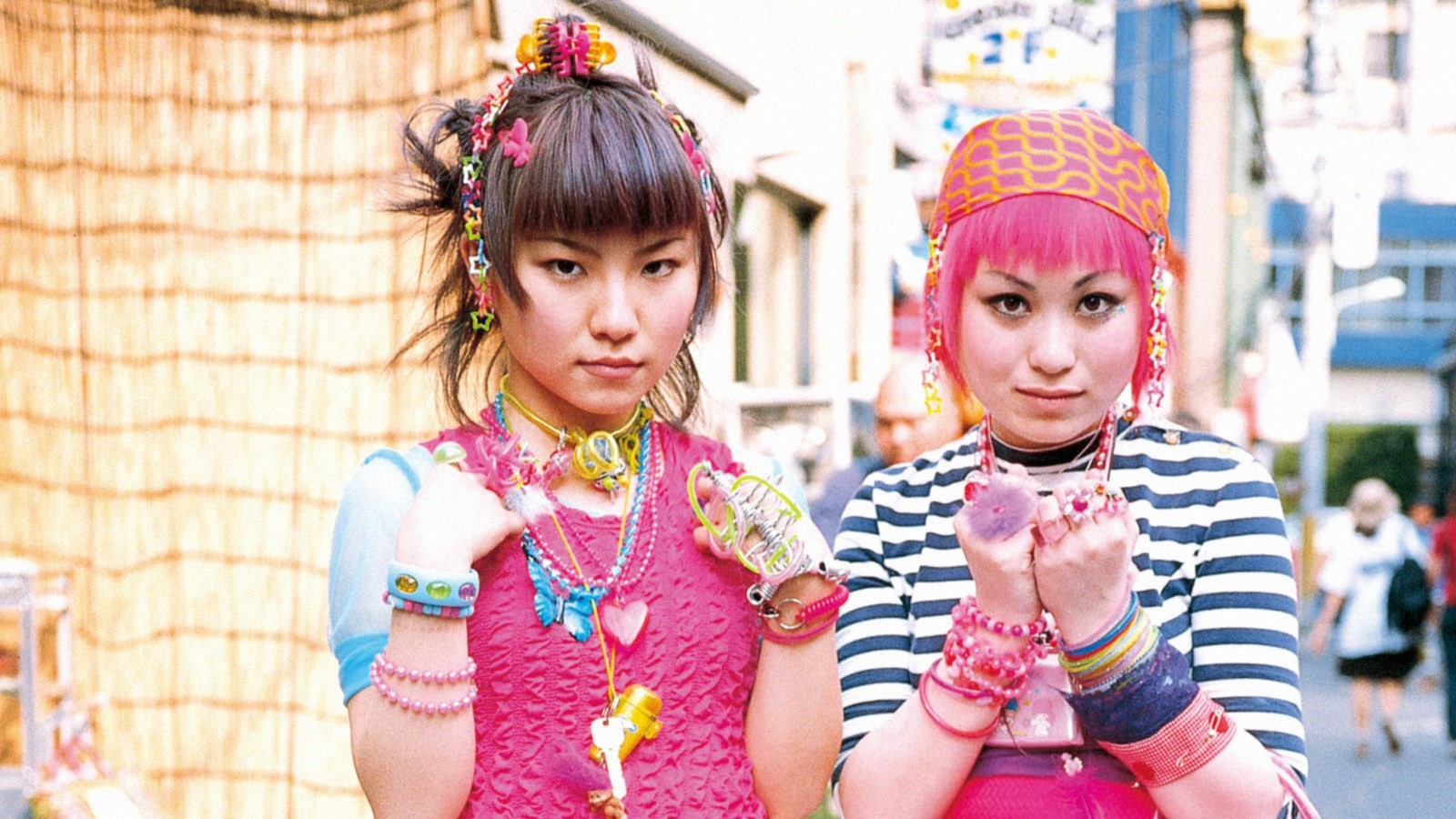The photo captures two young women, possibly preparing for an event, standing side by side and facing the camera. Both women have their arms raised, elbows tucked close to their bodies, and hands positioned near their shoulders. Their attire and accessories are elaborate and colorful. The woman on the right has striking pink hair adorned with a headband featuring small star shapes. She is dressed in a black and white striped shirt and wears numerous bracelets, including pink bead bracelets and silicone ones, along with rings. Her counterpart on the left has dark brown hair decorated with additional butterfly clips and similar star-shaped accessories. She is wearing a layered outfit consisting of a pink frilled shirt over a blue one, with numerous bracelets and necklaces, one of which features a heart, and another appears to have a key. The background reveals a busy outdoor setting in what appears to be China, with blurred buildings and signage, a brown curtain-like structure to the left, and a stand or cart in the bottom left corner. A woman dressed in white can be seen walking in the distance.